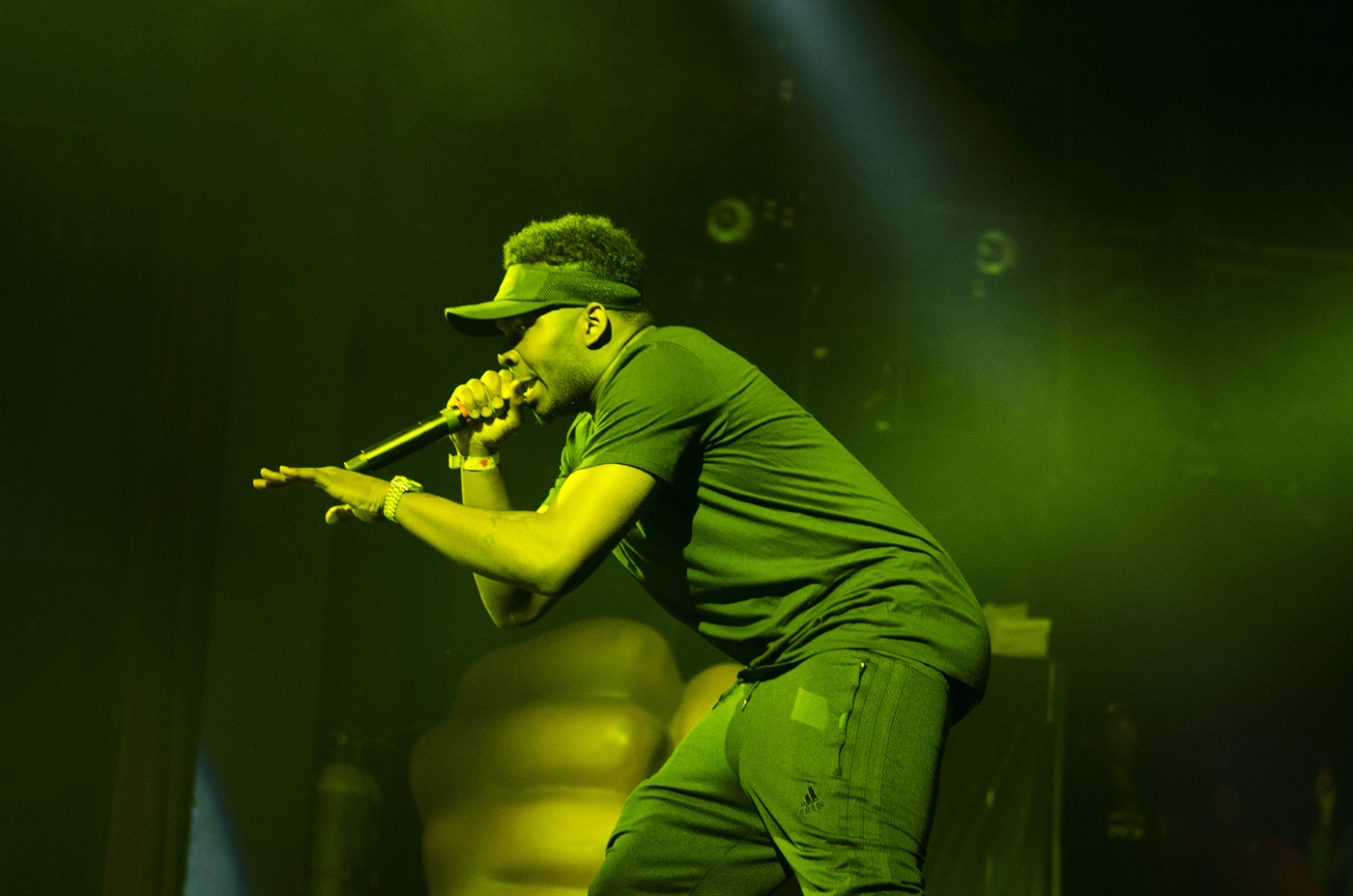The photograph captures a dynamic moment of a singer performing on stage, bent over slightly and looking towards the left side of the frame. Dressed in dark-colored pants featuring the Adidas logo and a matching short-sleeved shirt, the singer adds a sporty touch with a dark tennis visor atop their head, revealing a bit of their hair. The scene is bathed in a yellowish-green hue from the stage lights, casting a surreal tint over the entire image. The singer grips a black microphone in their right hand, bringing it close to their face, while their left arm extends outward, perhaps in a gestural expression accompanying their performance. A silver metal wristwatch adorns their left wrist, contrasting with the white wristband on their right. Behind the performer, a large black wall painted with bubble motifs and a striking 3D fist statue set an intriguing backdrop, complementing the intense focus of the on-stage action.